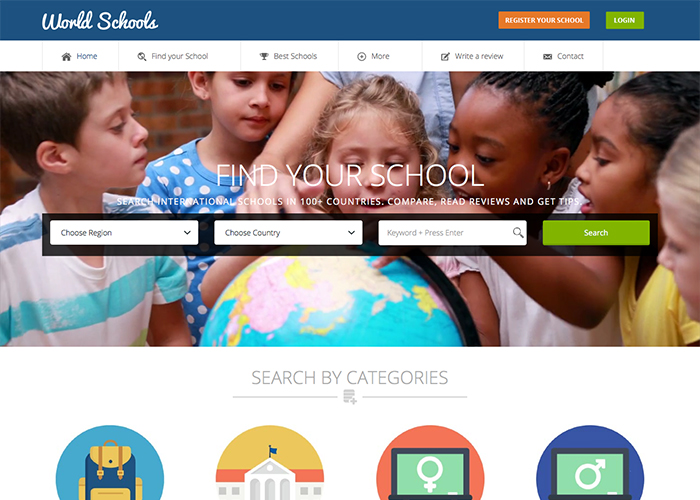The image depicts the homepage of the WorldSchools website, which focuses on international schools in over 100 countries. Users can compare, read reviews, and get tips on schools worldwide. At the top of the homepage, there are options to register a school and log in. The top menu bar includes the following sections, from left to right: Home, Find Your School, Best Schools, More, Write a Review, and Contact.

Dominating the center of the page is a prominent search area. In the background image, six children are gathered around a globe, some pointing and examining different regions. An adult, likely a teacher, stands behind one of the children, also pointing at the globe and engaging in a discussion.

The search bar runs across the middle of the background picture, allowing users to choose the region, country, and enter keywords before searching. At the bottom, users can search by categories, each represented by icons: a backpack, a schoolhouse, and universal symbols for female and male.